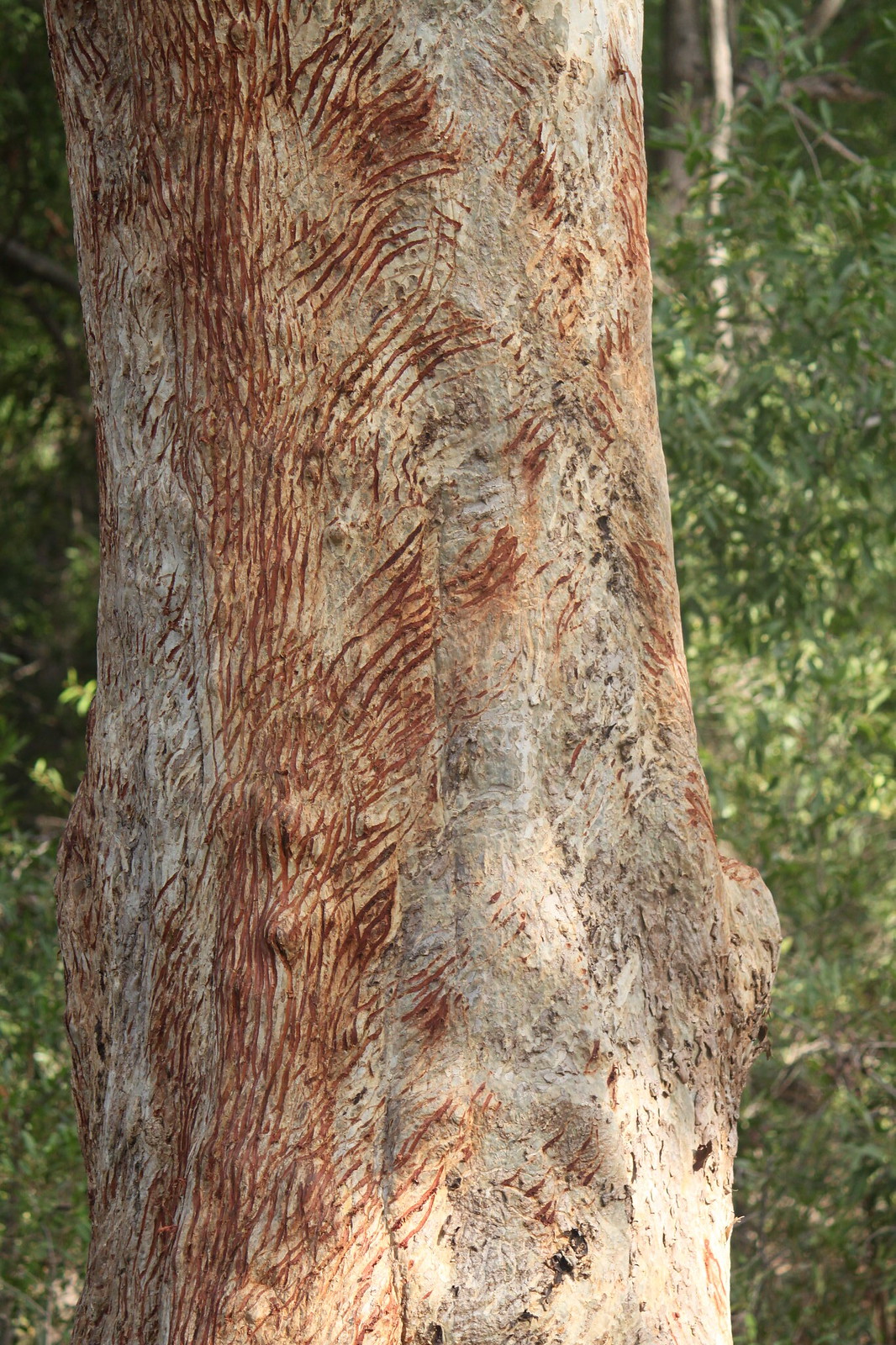This photograph is a vertical close-up shot of a tree trunk, showcasing its unique and striking appearance. The trunk is predominantly white to light beige in color, with the whiteness likely accentuated by sunlight. It features a distinctive texture marked by brown lines and scratch-like patterns that rise vertically along the trunk. These markings resemble claw marks, possibly from an animal, peeling away the outer layer and revealing a darker, reddish-brown inner layer beneath. The intricate scratches vary in direction, with some traveling vertically while others slant diagonally, often appearing in groups of four or five parallel lines. The tree trunk stands out as the primary focus of the image, framed by lush greenery on both sides, including shrubs, bushes, grass, and possibly leaves or flowers in the background. There are no branches visible in this tightly framed composition, emphasizing the detailed textures and natural patterns on the trunk itself.